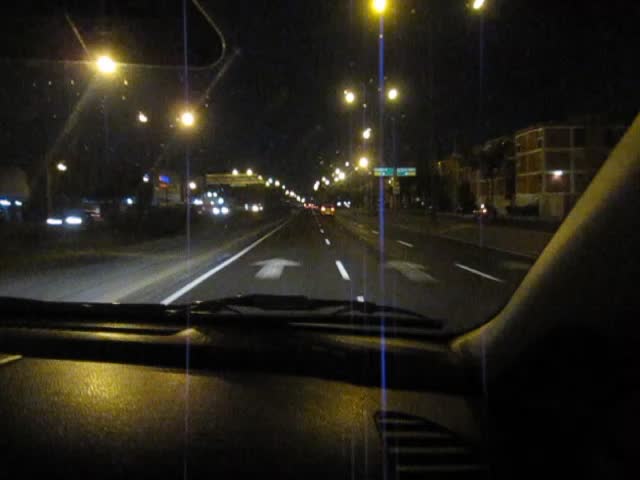This nighttime photograph, taken from the passenger seat of a car, reveals a color image of a divided highway with two forward-facing lanes marked by white arrows. The road is relatively empty with a few vehicles visible about a block ahead. To the left, a thick grass divider separates the lanes from oncoming traffic. A row of streetlights extends into the distance on both sides of the road, illuminating the scene against a dark night sky. On the right side of the image, a red brick apartment building with white cement lines is partially visible. Additionally, a green street sign with white writing stands out in the middle of the picture. Smaller splotches of light from street lamps dot the background, emphasizing the tranquil yet lively atmosphere of this urban night scene.